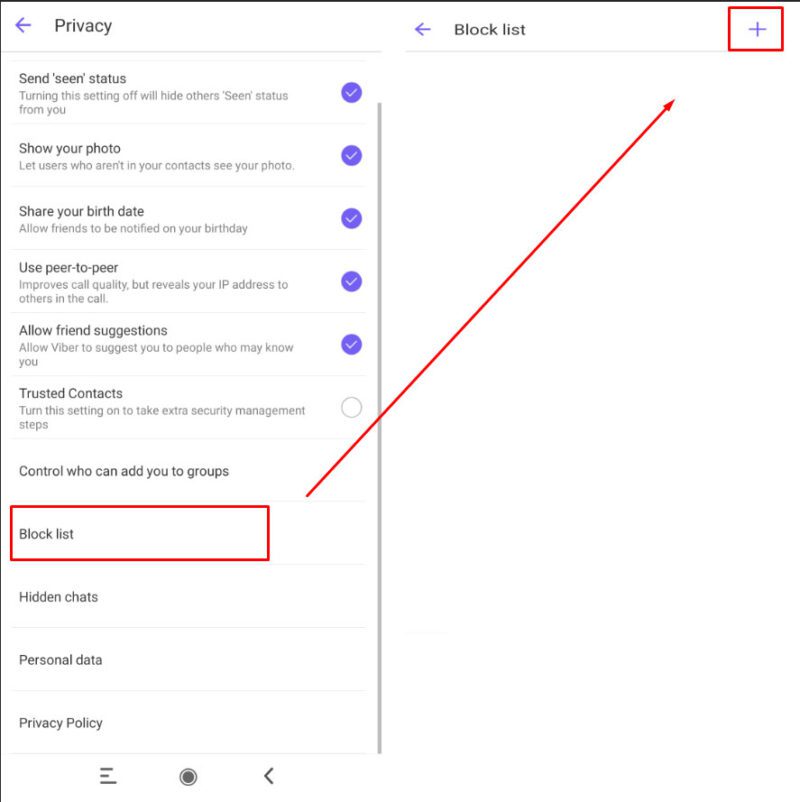The image showcases a close-up screenshot of a tablet or smartphone screen displaying a privacy settings menu. The text is presented in a way that requires a 200% zoom to be clearly legible, likely for privacy considerations. The menu includes several options with checkboxes, most of which are selected. These options are:

- "Send scene status" (checked)
- "Show your photo" (checked)
- "Share your birth date" (checked)
- "Use peer-to-peer" (checked)
- "Allow friend suggestions" (checked)
- "Trusted contacts" (not checked)
- "Control who you can add to your group"

In bold red text, the menu prominently features "Block list," next to which there is a large arrow pointing to a plus sign located at the top right corner of the screen. This is followed by options for "Hidden chats," "Personal data," and "Privacy policy," with a left-pointing arrow situated immediately before "Block list."